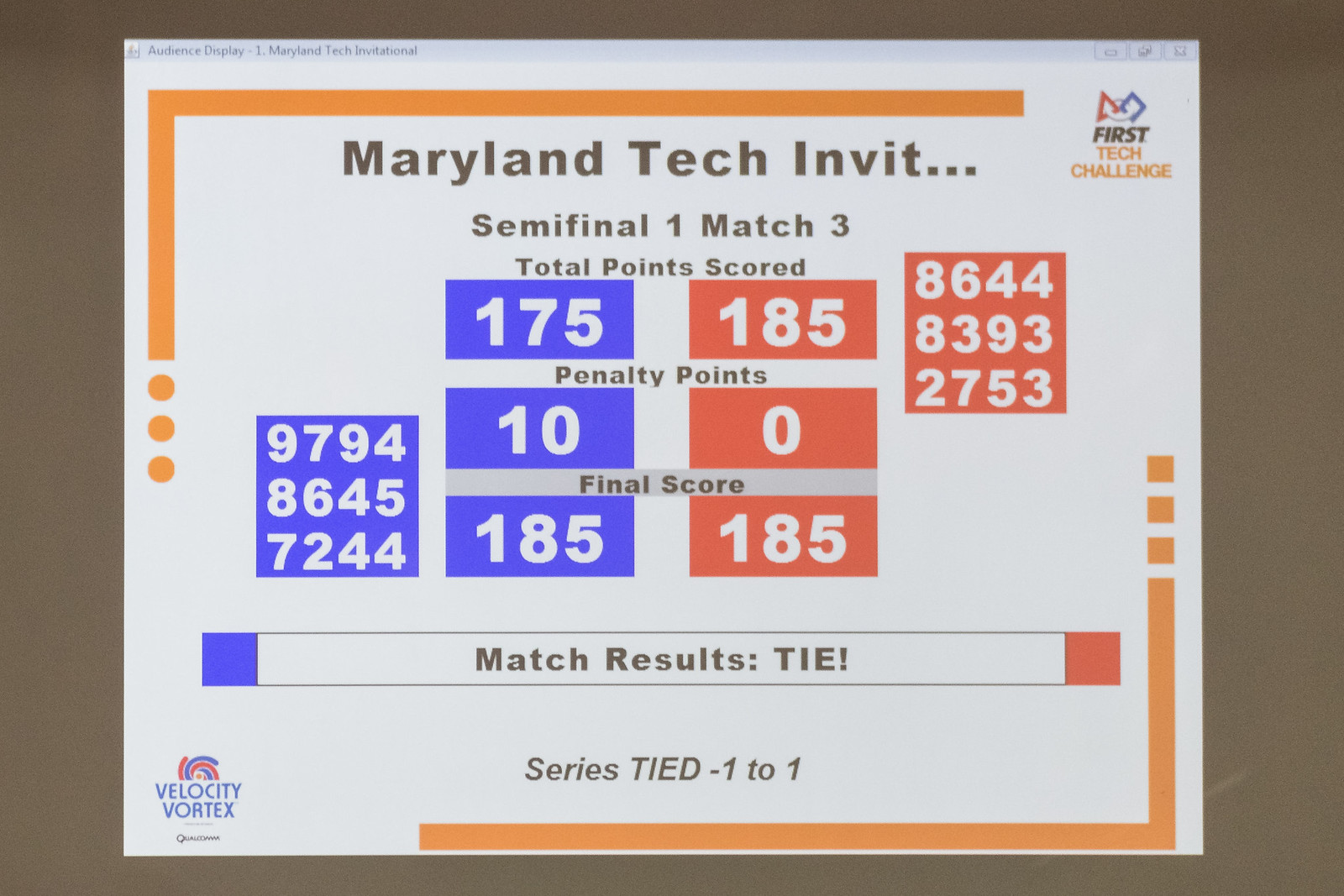The image shows a computer screen displaying a slide, likely from a presentation or scoreboard, with a white background and multicolored text in blue, red, yellow, and black. At the top, the slide reads "Maryland Tech Invitational" and at the upper right corner, "First Tech Challenge." The central part of the screen includes the heading "Semi-Final One, Match Number Three," followed by "Total Points Scored." 

On the left, within a blue background, it states "Total Points Scored: 175." To the right, within a red background, it reads "Total Points Scored: 185." Below these scores are the penalty points: "10" on the left and "0" on the right, leading to a final tied score of "185 to 185." Beneath these details, the slide announces "Match Results" and emphatically states "TIE!" in all capital letters. At the very bottom, it reads "Series Tied 1 to 1."

Additionally, on the left side of the screen within blue boxes, there are numbers "9,794," "8,645," and "7,244." Correspondingly, on the right side within red boxes, there are numbers "8,644," "8,393," and "2,753."